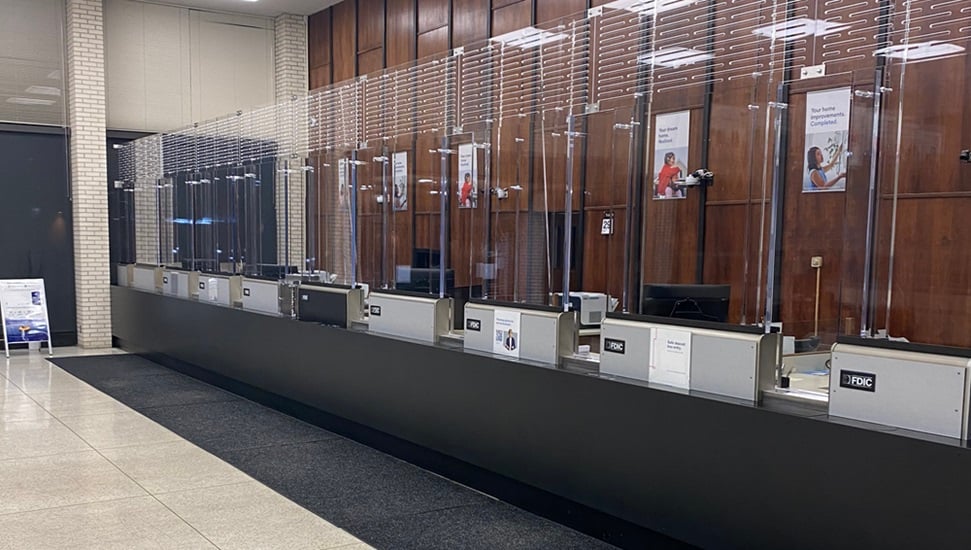The interior image depicts a spacious, public-access building that is evidently a bank, identifiable by the multiple teller stations adorned with FDIC stickers. The scene is devoid of people and features a sleek, industrial design. The customer area is defined by a long gray carpet in front of the teller stations, contrasting with the white and dark gray marble flooring elsewhere. The right side is lined with white brick pillars and either white walls or shades above the windows, while the rear wall is distinguished by its dark brown wood paneling with a potential door just right of the center. Seven teller stations, equipped with clear glass or plexiglass panes for customer interactions, remain unoccupied, with small openings for transactions. Above and behind the stations, various posters are visible, though their content remains unreadable. Vertical reflections of ceiling lights are scattered on the glass panes, adding to the room’s bright ambiance. Far in the background, a sandwich board sign can be seen, although its details are unclear. The teller stations are equipped with technological devices like computers and printers, enhancing the functionality of this evidently busy banking environment.